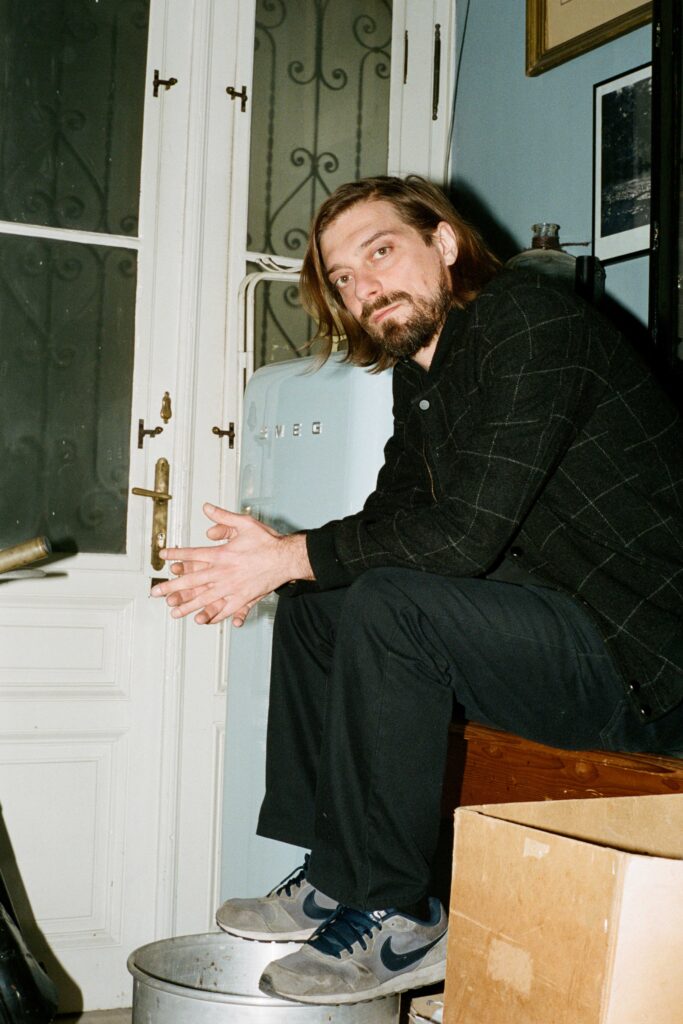The photograph captures a young man with long, wavy brown hair, a mustache, and a short beard, sitting on a wooden platform or desk just inside or outside a doorway. He has a serious expression on his face as he looks at the camera, his hands clasped in front of him. He is dressed in a black long-sleeved, plaid jacket with faded white stripes, long black pants, and gray Nike sneakers with green Swoosh logos and green shoelaces. His feet rest on the rim of a silver metal bucket, and to his side is a brown cardboard box. Behind him, there is an old-fashioned, curved light blue refrigerator and a white door with gold hinges and a frosted window. The wall next to him is painted light blue and adorned with some photographs.